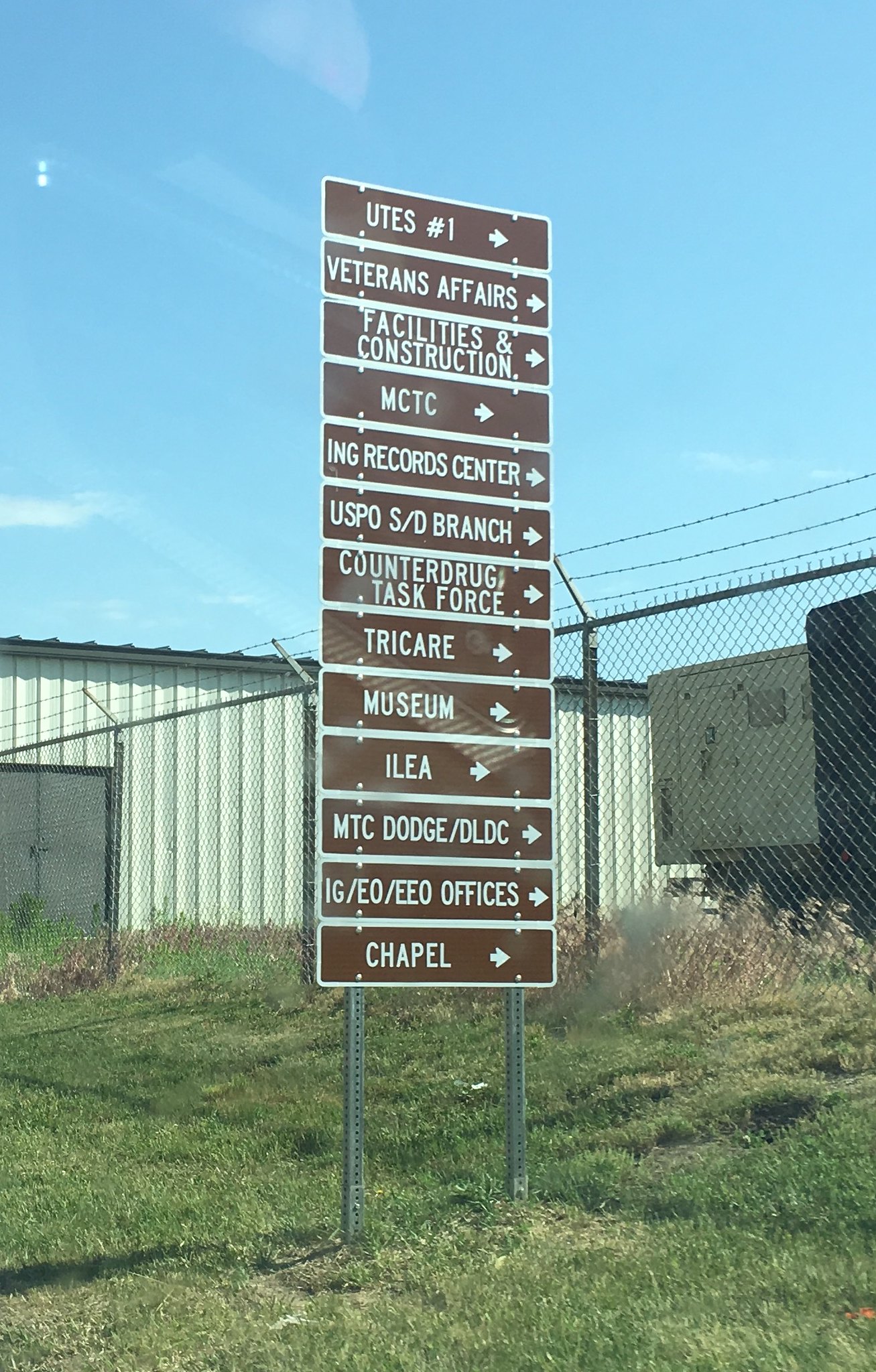This image features a large directional sign located on a grassy roadside, likely indicating destinations within a military base. The sign is mounted on two silver poles and consists of several dark brown rectangular panels with white lettering and white arrows pointing to the right. The text on the panels reads: UTES #1, Veterans Affairs, Facilities and Construction, MCTC, ING Records Center, USPOS/D Branch, Counter Drug Task Force, TRICARE, Museum, ILEA, MTC, DODGE/DLDC, and Offices & Chapel.

Behind the sign, the sky is a clear, vibrant blue extending across the top half of the image. Midway down, there is a corrugated steel building in a creamish color, featuring a black steel door on the left side, running about three-quarters across the image. To the right of the building, there appears to be a lighter-colored trailer or another structure.

A silver chain-link fence topped with barbed wire runs horizontally near the base of the sign, with tall brown dead grass in front of it and neatly cut grass immediately surrounding the sign. There are no people visible in the photograph, emphasizing the stark and orderly setting typical of a military environment.